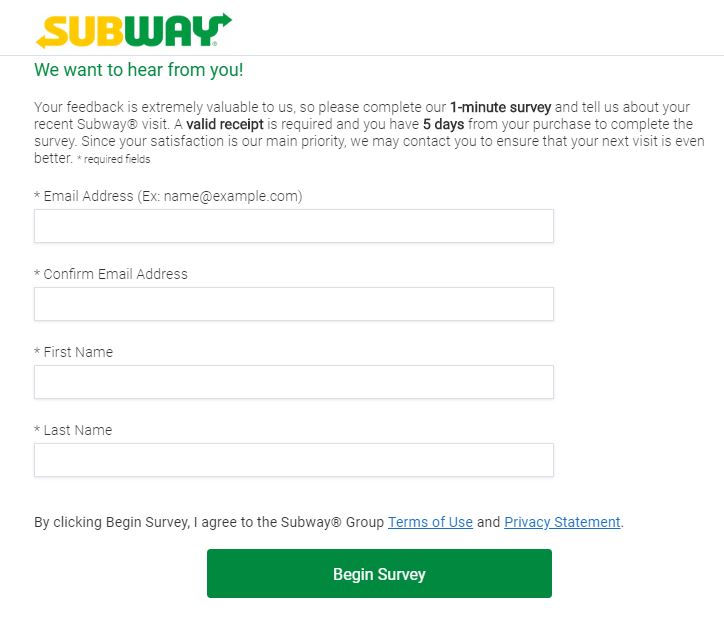The image captures a Subway feedback request form prominently displayed on a clean, white background. It encourages customers to participate in a one-minute survey to share their recent dining experiences. The form highlights that a valid receipt is required and must be used within five days of the purchase date. It appears that the form was received after placing an order online, and includes fields for email, confirmation of the email, first and last name, and an option to upload a picture of the receipt.

The form emphasizes the significance of customer satisfaction and mentions the possibility of follow-up contact to enhance future visits. Positioned towards the bottom is a green "Begin Survey" button, along with a statement indicating that by clicking the button, users agree to Subway's terms of use and privacy statement.

The iconic Subway logo is prominently featured at the top, with its distinctive design: the word "Sub" in yellow and "Way" in green, complemented by arrows at the ends of the 'S' and 'Y'. The text on the form is in standard black, maintaining clarity and readability against the white backdrop.